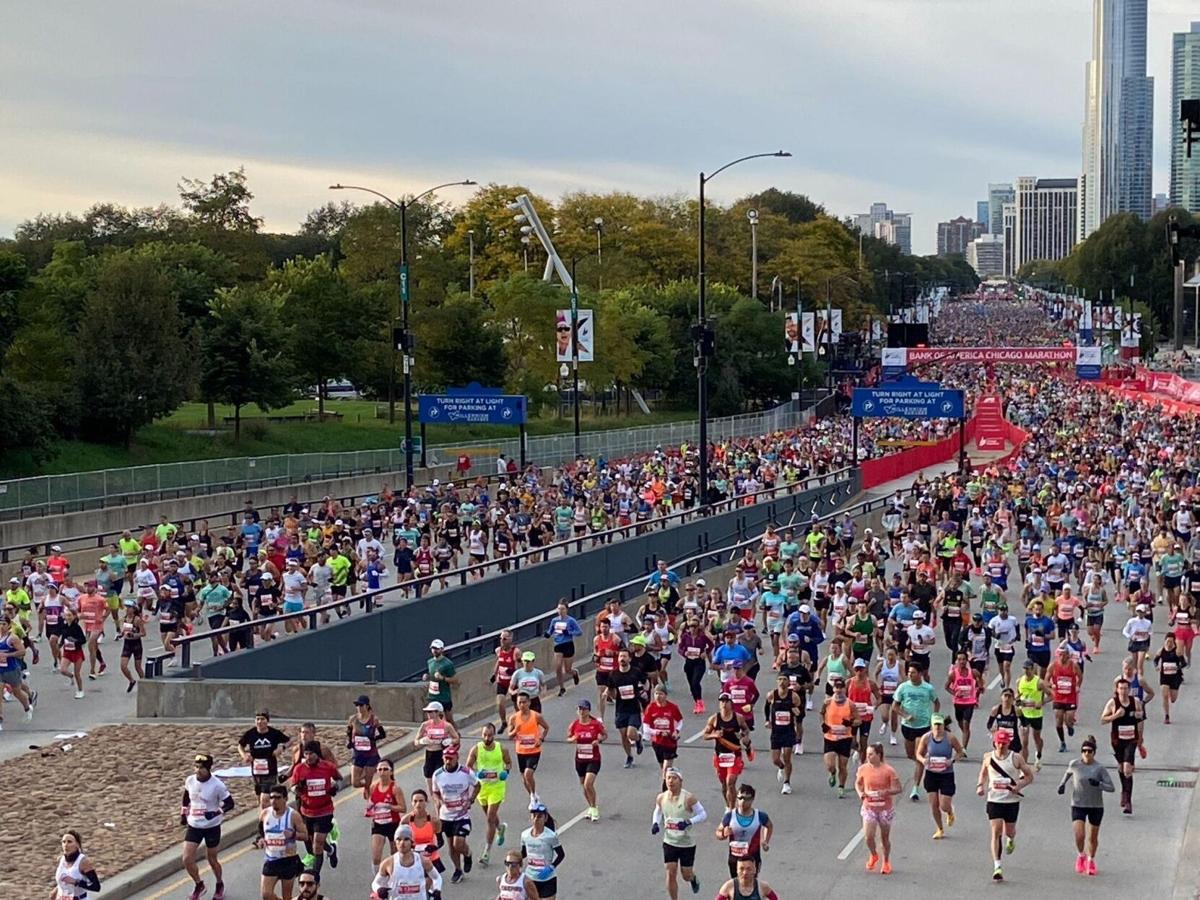The image captures the exhilarating start of the Bank of America Chicago Marathon, with thousands of runners packed tightly into a major street that is elevated above a corridor of cars below. The sky overhead is grayish, providing a dramatic backdrop to the scene. In the far right background, the skyscrapers of Chicago's iconic skyline are visible, reinforcing the urban setting of this renowned race. 

In the middle background, a large red banner prominently displays "Bank of America Chicago Marathon," confirming the event location. The street is a sea of motion, with runners wearing a variety of brightly colored attire, including a notable amount of orange, green, and black. Each participant wears a race number on their chest, indicating they are all competing. The scene appears to be near the starting point of the marathon, as the density of runners increases further back towards the city, forming a densely packed river of people surging forward. 

To the left of the runners, there's a parkway filled with dense foliage, providing a contrasting natural boundary to the urban race route. The elevated vantage point of the photograph suggests that the camera might have been positioned on a platform, offering a commanding view of the massive crowd as they embark on their marathon journey.